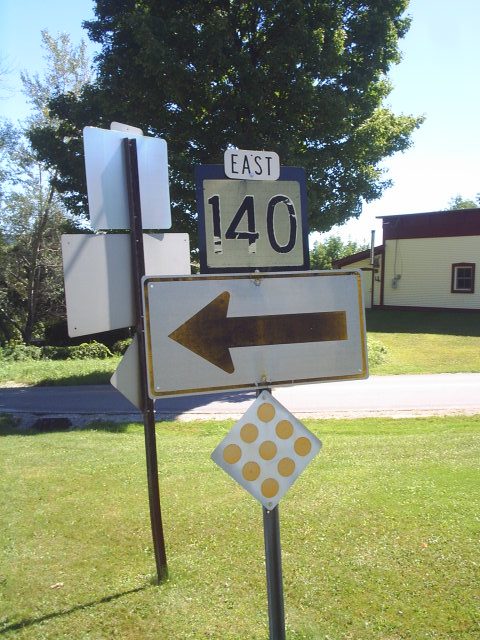This image showcases two sets of street signs mounted on a sturdy silver metal pole, situated in a grassy area beside a small road. The prominent sign facing forward at the top features a small white plaque with black letters indicating the direction "EAST." Below it, a larger silver sign bordered in blue displays the route number "140" in white numerals. Following this, there is a sizeable white sign with a yellowish-brown border, revealing a left-pointing arrow in brown with a yellow tint. Further down the pole, a diamond-shaped sign is adorned with nine yellow circles.

In the background to the left, there is another set of street signs identical in shape and configuration to the ones described. The area is lush with greenery, and a vivid blue sky stretches above. Dominating the scene is a large tree flourishing with vibrant leaves, accompanied by a smaller tree that is sparsely leafed. Behind this arboreal setting stands a well-maintained beige structure with a clean, new-looking brown roof.